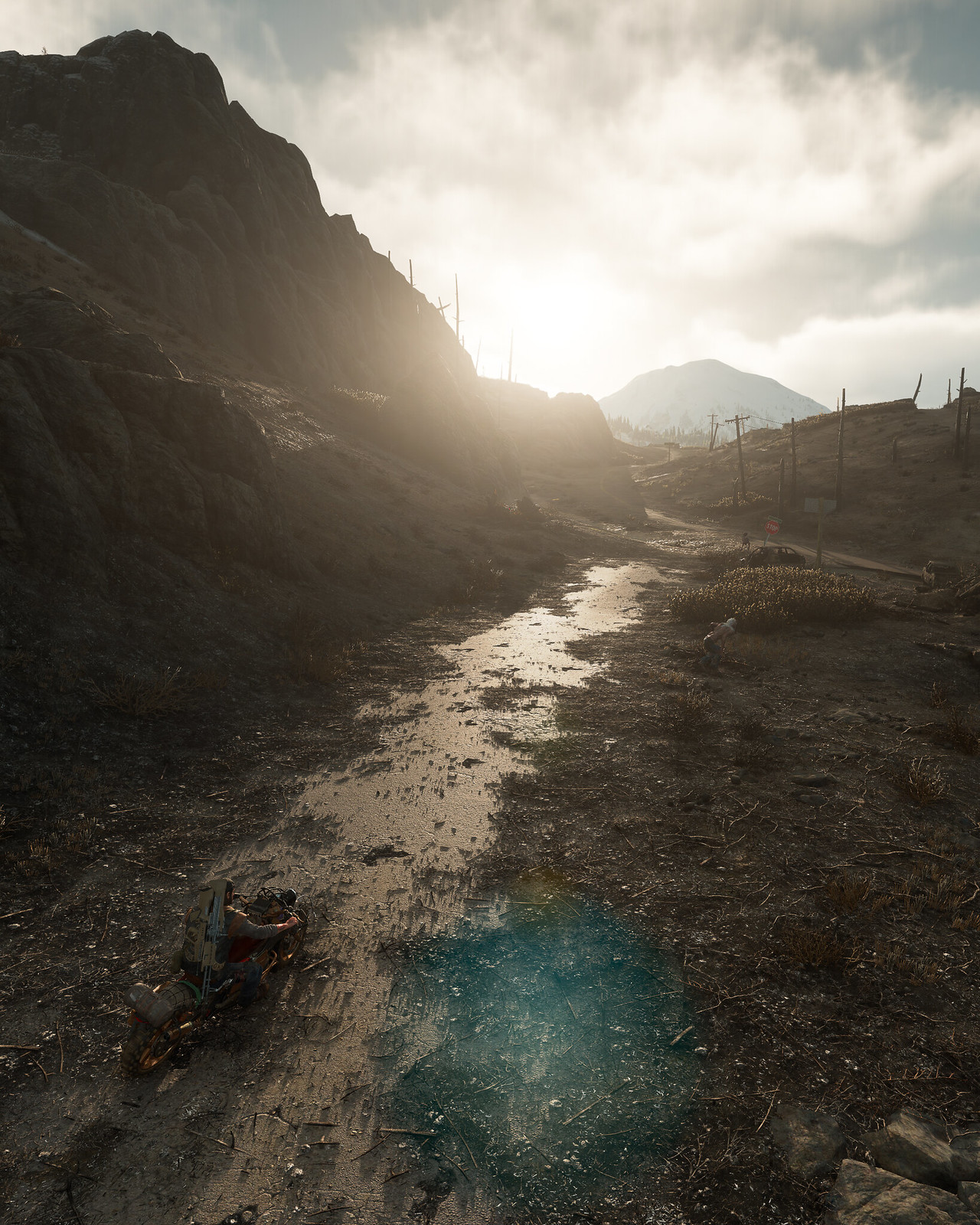This outdoor photograph features a rugged, muddy trail snaking through a craggy landscape dominated by a mountain range on the left side. The horizon is graced by a larger, shadowy mountaintop, with the sun peeking over it, casting a bright but diffuse light through a gray sky mottled with white clouds. The early morning light illuminates the wet, rocky pathway, making it appear shiny. Sticks and sparse vegetation punctuate the muddy expanse, contributing to a scene of barren beauty.

To the right of the trail, there's a clearing marked by scattered debris and faint green plants. A figure crouches in the distance alongside an abandoned black car. Further along, telephone poles punctuate the landscape, enhancing the sense of desolation.

In the foreground, a man on a dark motorcycle, possibly wearing a backpack and brown fatigues, navigates the rough path. The motorcycle's orange spokes add a splash of color to the otherwise earthy palette. The scene might seem a bit surreal, possibly due to an unrealistic bluish watermark to the right of the trail, hinting at either artificiality or a reflection. This element gives a subtle, unique touch to the overall composition, blending the stark natural environment with an air of mystery.